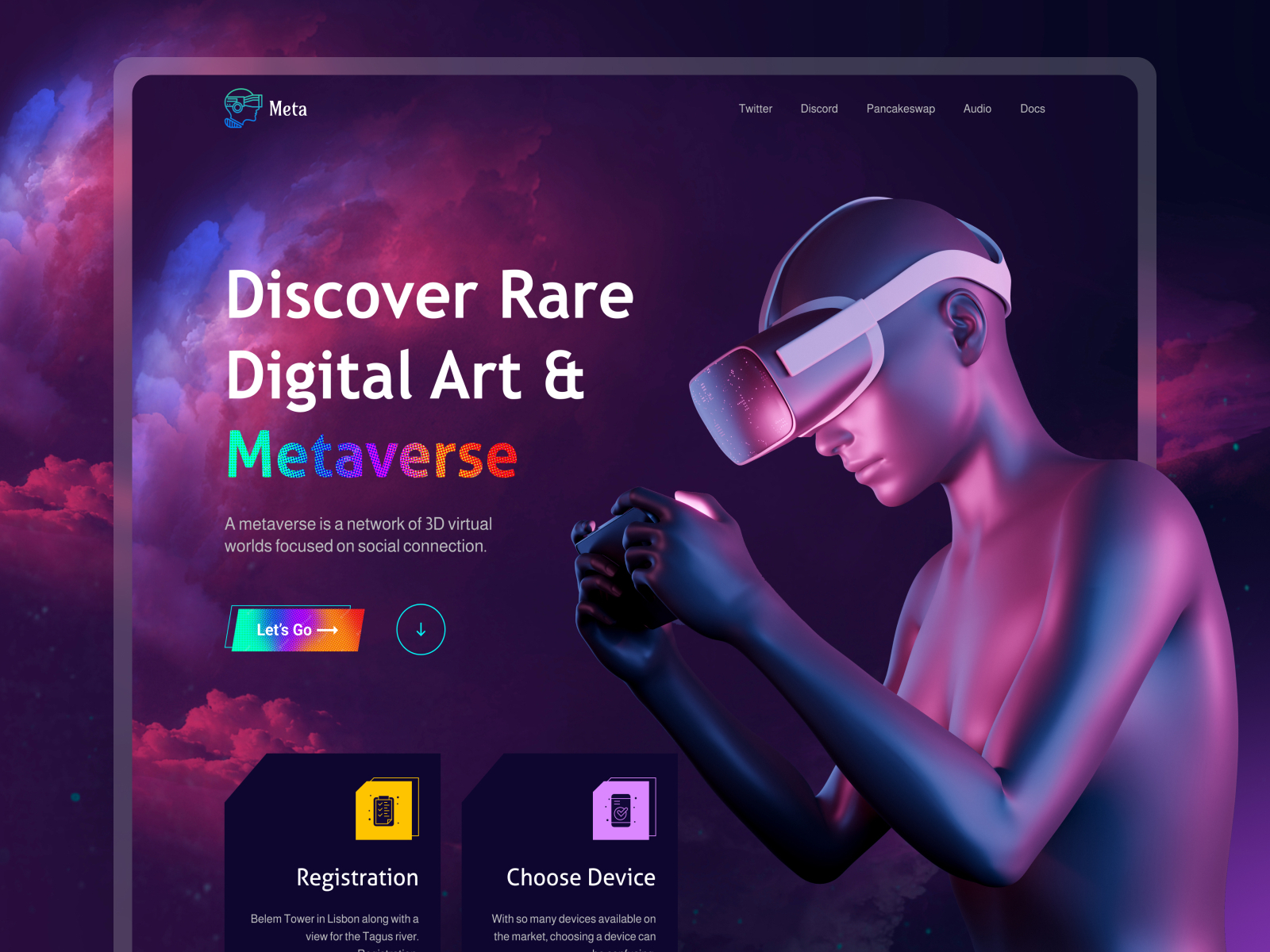This advertisement for Meta's website features a vivid, stylized background composed of dark, purple, blue, red, and pink cloudscapes. Superimposed on this backdrop is the website interface, prominently displaying the Meta logo in the top left corner. An icon of an individual wearing an Oculus VR headset is also placed near the Meta logo.

To the right of the logo, clickable icons for various linked pages, including Twitter, Discord, PancakeSwap, and AudioDocs, are neatly arranged. The primary section of the webpage showcases the phrases "Discover Rare Digital Art" and "Metaverse," indicating the platform's focus. Beneath "Metaverse," it describes the network as consisting of three virtual worlds centered on social connection.

Further down the page, users are prompted to explore options for downloading, registering, and choosing a device, along with settings for individual device setup. Adjacent to these instructions, there is a detailed 3D-rendered image of a mannequin-like human figure. This figure, devoid of distinguishing features, is depicted holding a VR controller with both hands and wearing a VR headset.